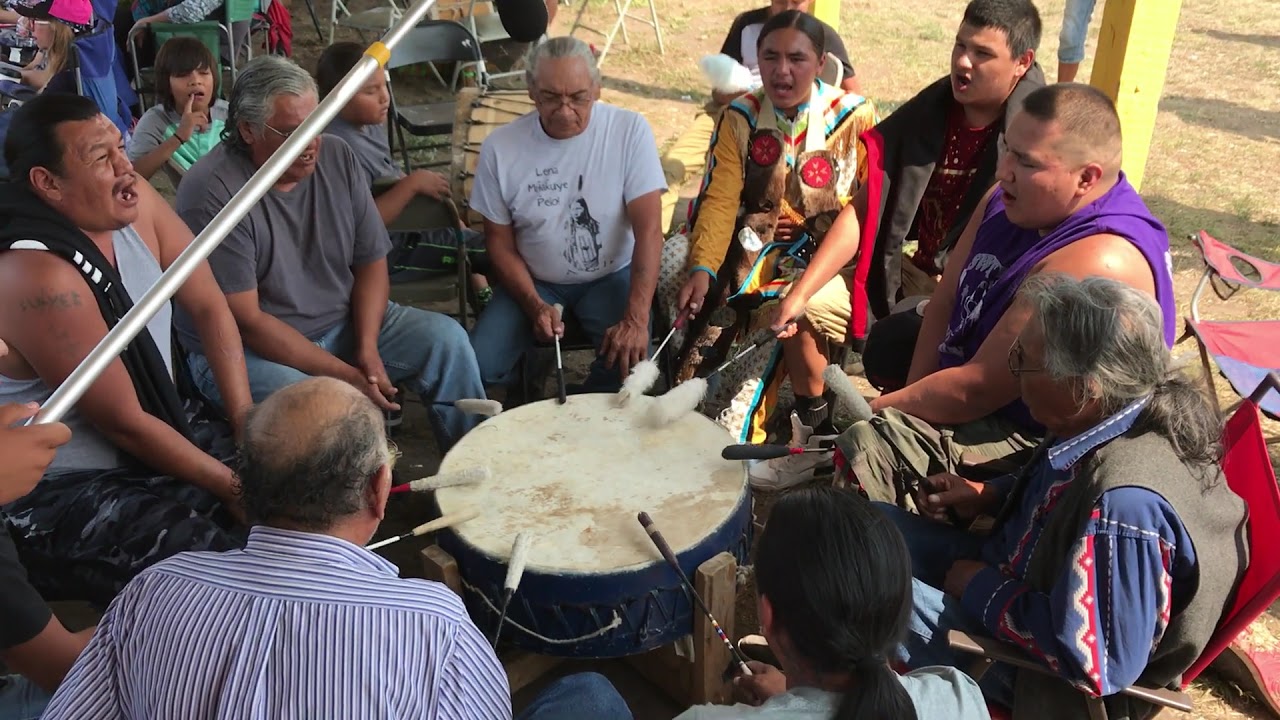This vivid outdoor photograph captures a group of ten Native American men seated in a circle, engaged in a traditional drumming ceremony. The image, taken during daylight hours with natural light, is shot from a slightly elevated angle, revealing the details of the scene below. The setting appears shaded, likely due to a large yellow wooden post supporting an overhead cover, with sunlight streaming in from the right. The men, ranging from younger to older, with dark or grayed hair, exhibit a rich variety in attire—some wearing jeans and t-shirts, one in a collared shirt, and another dressed in traditional Native American attire. 

At the center of the group is a large blue drum with a white canvas or leather surface. Each participant holds a unique drumstick, some adorned with white feathers or poofy heads, and others in black or plain white. They strike the drum in unison, mouths open as if chanting or singing, contributing to the ceremonial atmosphere. The background features browned grass, suggesting an outdoor setting during a dry season. Folding chairs are visible in the upper left portion, hinting at preparation for a larger gathering or audience.